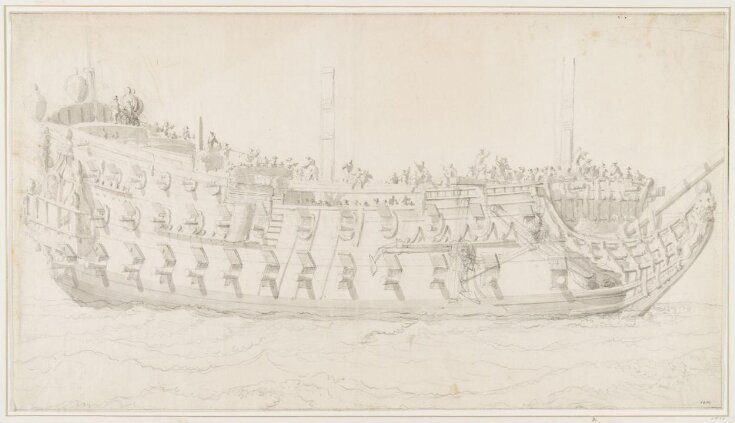This detailed black-and-white graphite sketch portrays an ancient warship sailing on the water, facing right. The ship, resembling old pirate or cargo ships, features an intricate hull with two main observable decks. Along the side, there are about 12 to 15 cannons protruding through open hinged doors, arranged in three distinct rows. The delicately drawn waves suggest movement in the water.

Men are scattered across the ship's top deck, actively working, hinting at the ship's bustling nature. On the left side of the boat, decorative elements are visible on the stern, while on the far right, a long bowsprit extends forward, reinforcing the ship's ancient build. Two tall masts, though void of sails, stand prominently in the center and towards the right side of the vessel. The aged, creamy paper and the sketch's faint lines, along with a nearly indecipherable signature in the bottom right corner, contribute to its antique aesthetic.